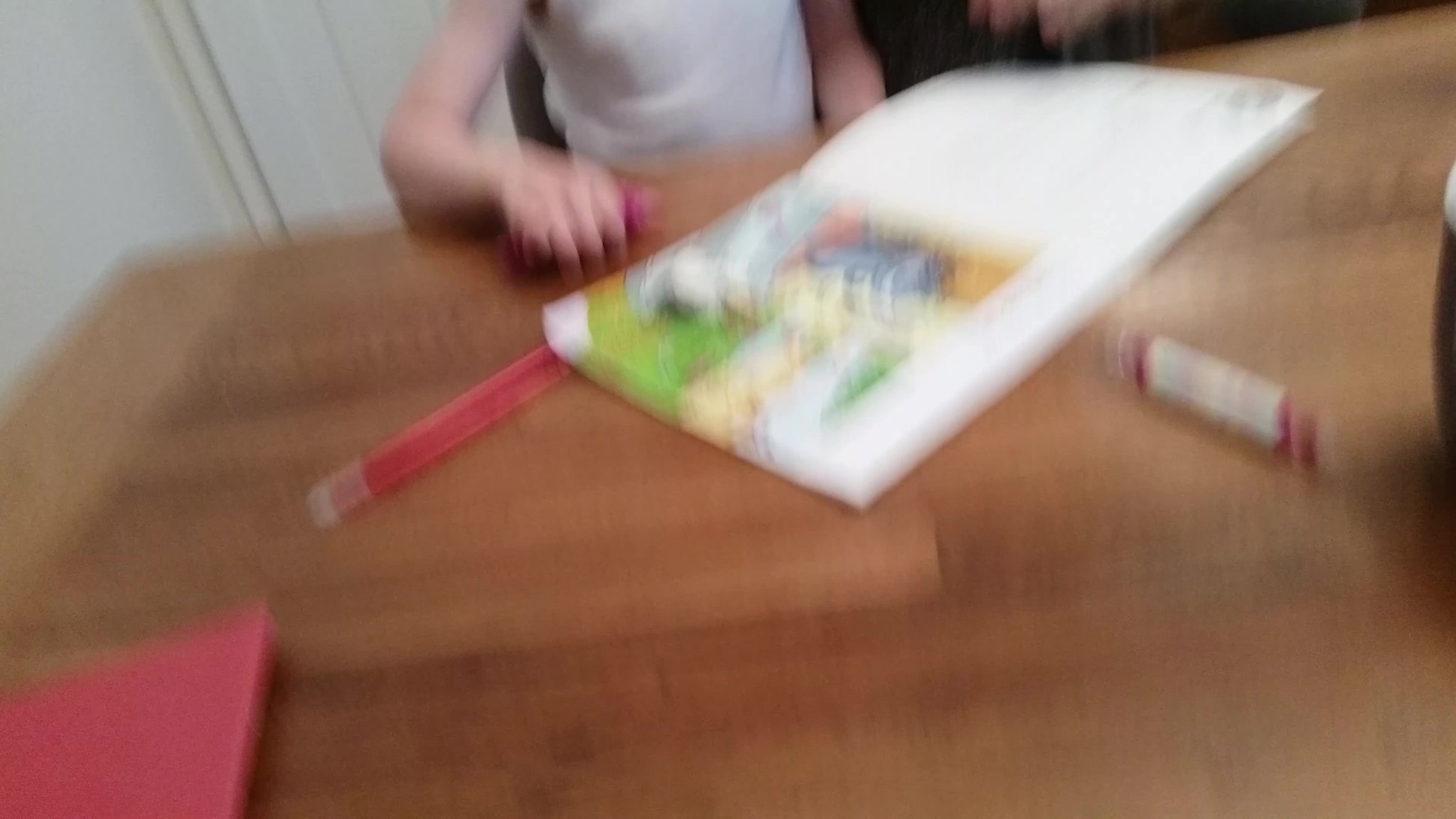An out-of-focus photograph depicts a wooden table adorned with a large, open coloring book. The coloring book is noticeably wider and more spacious than a standard book, featuring various sections meant for coloring. Seated at the table is a young child, whose face is not visible, making it difficult to determine their gender, but their age appears to be around six years old. The child clutches a fistful of what appears to be crayons, though the blurriness makes it hard to be certain. Other than the coloring book and the handful of crayons, the table has a few indistinct objects scattered around. In the bottom corner of the image, a red folder is partially visible, also placed upon the wooden tabletop.